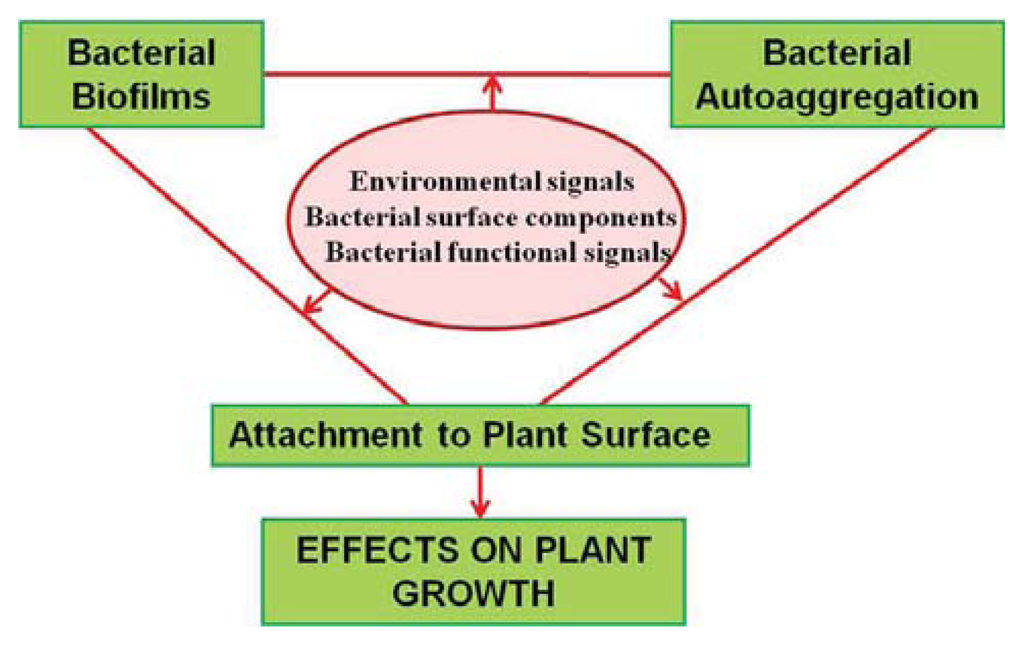This diagram, set against a white background, depicts the interactions of bacterial biofilms and auto-aggregation in relation to plant growth, using green text boxes and a central red-trimmed oval. In the upper left corner, a green box with black writing is labeled "Bacterial Biofilms," while in the upper right corner, another green box is labeled "Bacterial Auto-Aggregation." These boxes are connected to a central red oval, which contains the text "Environmental Signals, Bacterial Surface Components, Bacterial Functional Signals." Red lines and arrows link this central oval to the upper text boxes and a lower green box labeled "Attachment to Plant Surface." Further down, another arrow leads to a final green box that says "Effects on Plant Growth." This flowchart is organized in a downward-pointing triangle, illustrating a step-by-step process of bacterial interactions affecting plant growth.